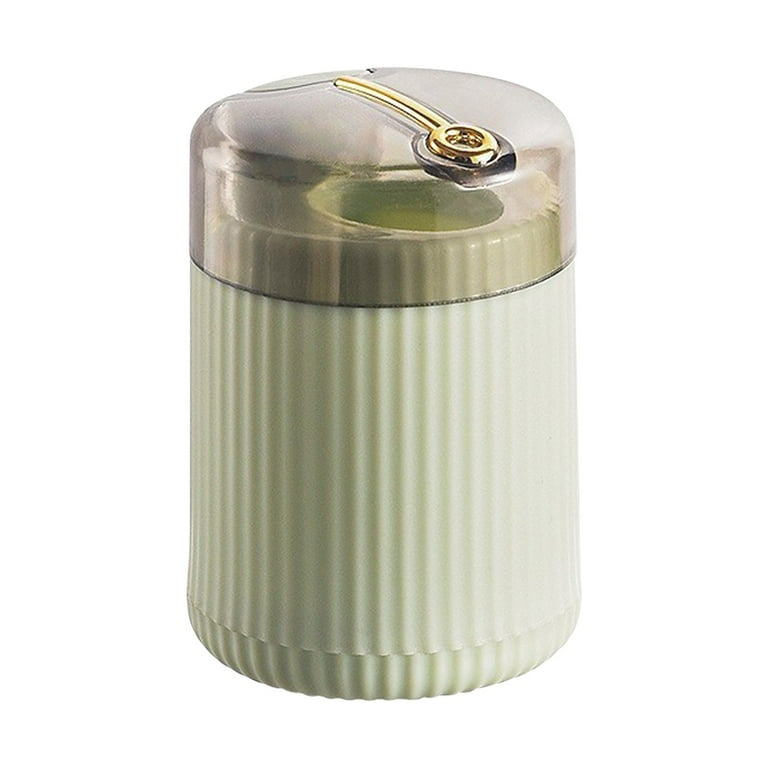The image depicts a highly designed cylindrical container, which appears to serve as a holder for liquids or spices, potentially suitable for tabletop display. The body of the jar is cream-colored with a ribbed or fluted texture running vertically around it. The container features a translucent lid with a brownish-golden tint, through which a small round opening at the top of the jar is visible. The lid is crowned with a small gold piece or spout that seems functional, possibly for dispensing the contents. The container exudes a refined design aesthetic, visible against a neutral white background.